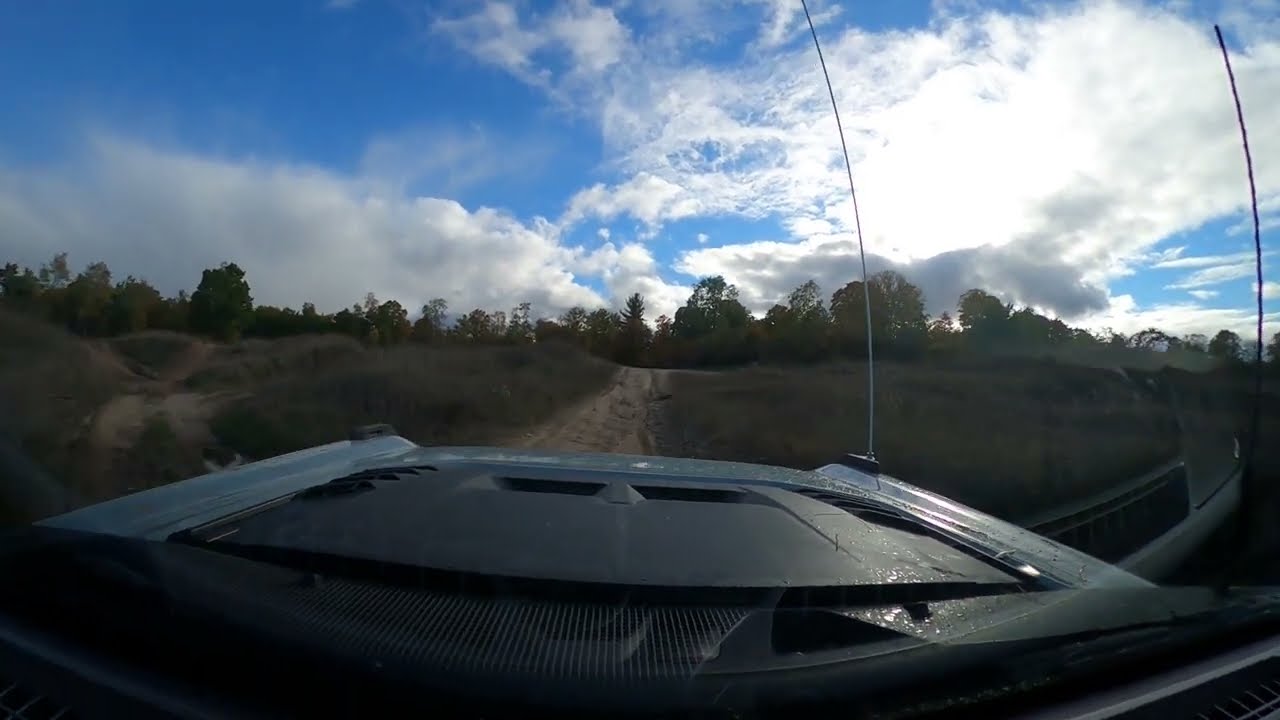This wide rectangular image captures the perspective from within an open-top, possibly ATV-like vehicle with a shiny black and light blue hood, dotted with droplets. The hood features two vertical antennas on its right side and visible vents. The vehicle is navigating a rutted, gray dirt path that gives the impression of slight bumpiness but remains mostly flat. The path converges toward the center of the image, with another track veering off to the left.

Flanking the dirt road are tall weeds, grasses, and a browny-green field, leading to a dense line of tall, leafy trees stretching across the horizon. The upper half of the picture is dominated by a vibrant blue sky, interspersed with feathery white and denser gray clouds, suggesting a dynamic weather setting. This detailed view offers a vivid snapshot from the driver or front passenger’s seat, emphasizing the rugged yet scenic journey through a grassy terrain.